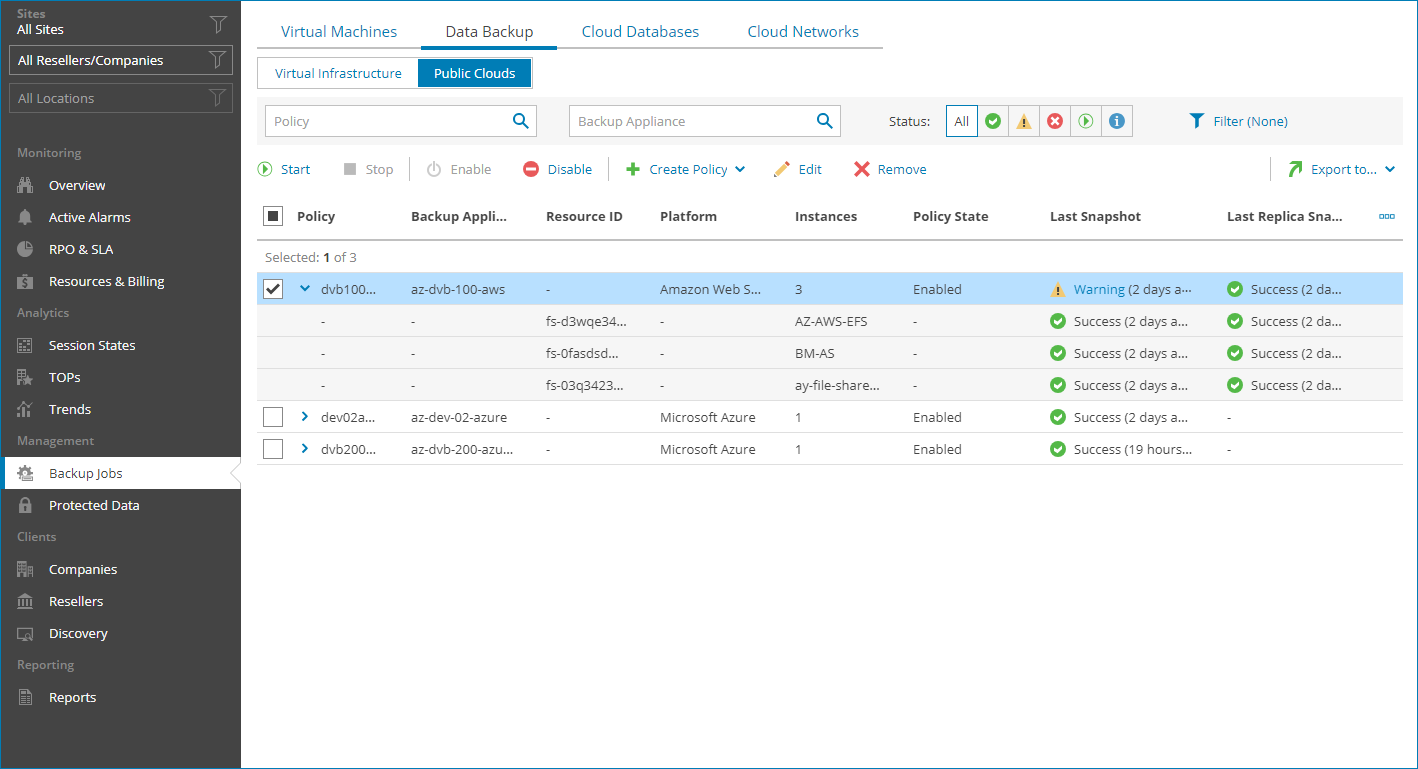The image displays a detailed interface of a site with an organized sidebar on the left. The sidebar features several filter options including one for all resellers and companies, which allows users to narrow their search by location. Below this, there is a 'Monitoring' section with multiple subsections such as Overview, Active Alarms, RPA and SLA, and Resources and Billing.

Further down, the 'Analytics' section includes Session States, TOPS, and Trends. The 'Management' section follows, offering options for Backup Jobs, Failover Plans, and Protected Data. There is also a 'Clients' section focusing on Companies, Resellers, and Discovery. Finally, a 'Reporting' section is available, containing Invoices and Reports.

The main screen to the right is currently displaying information related to backups, as indicated by the selected 'Backup Jobs' option under the 'Management' section. This part of the interface shows different elements such as Computers, Virtual Machines, Data Backup, Cloud Databases, and Microsoft 365 Objects. Users can utilize a variety of search and filter options to refine their data and can create policies for tasks like performing specific backups or taking snapshots of Azure images at scheduled times.